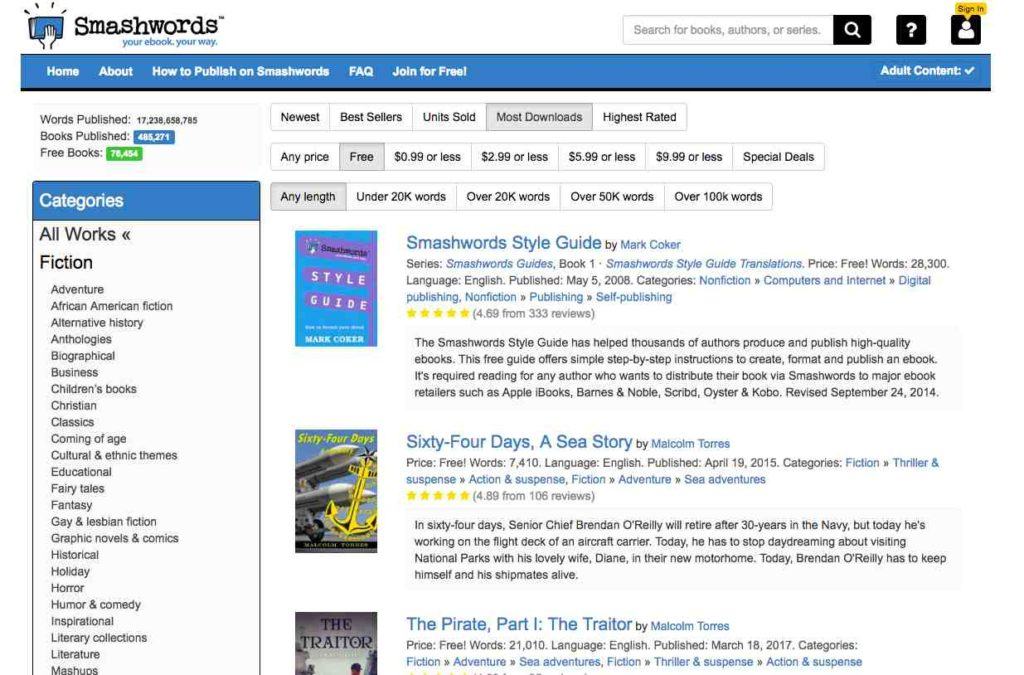This image is a screenshot from the Smashwords website. Dominating the center of the image is a hand holding a closed book, symbolizing control over one's own e-book. Beneath the Smashwords logo, the tagline "Your e-book, your way" is displayed in small blue print.

At the top of the page, there is a lengthy, narrow blue rectangle bordered in black. This contains white text with navigational links, including "Home," "About," "How to Publish on Smashwords," "FAQ," "Join for Free," and on the far right, "Adult Content" with a check mark indicating it has been selected.

On the left side of the image, a sidebar categorizes options for navigation, such as "All Works" and "Fiction." At the very top of this section, there are metrics displayed: "Words Published" with a large number, "Books Published" reporting 485,271, and "Free Books" at 76,454.

Moving towards the right, there are several more clickable listings like "Newest," "Best Sellers," "Units Sold," and "Most Downloads," with "Most Downloads" currently selected. Other filters further refine the search, such as "Free" and "Any Length," which are also chosen. Additional options include "Highest Rated," along with various price categories like "99 cents or less," "$2.99 or less," "$5.99 or less," "$9.99 or less," and "Special Deals."

This detailed layout allows users of the Smashwords platform to easily navigate and filter through the extensive library of e-books available on the site.